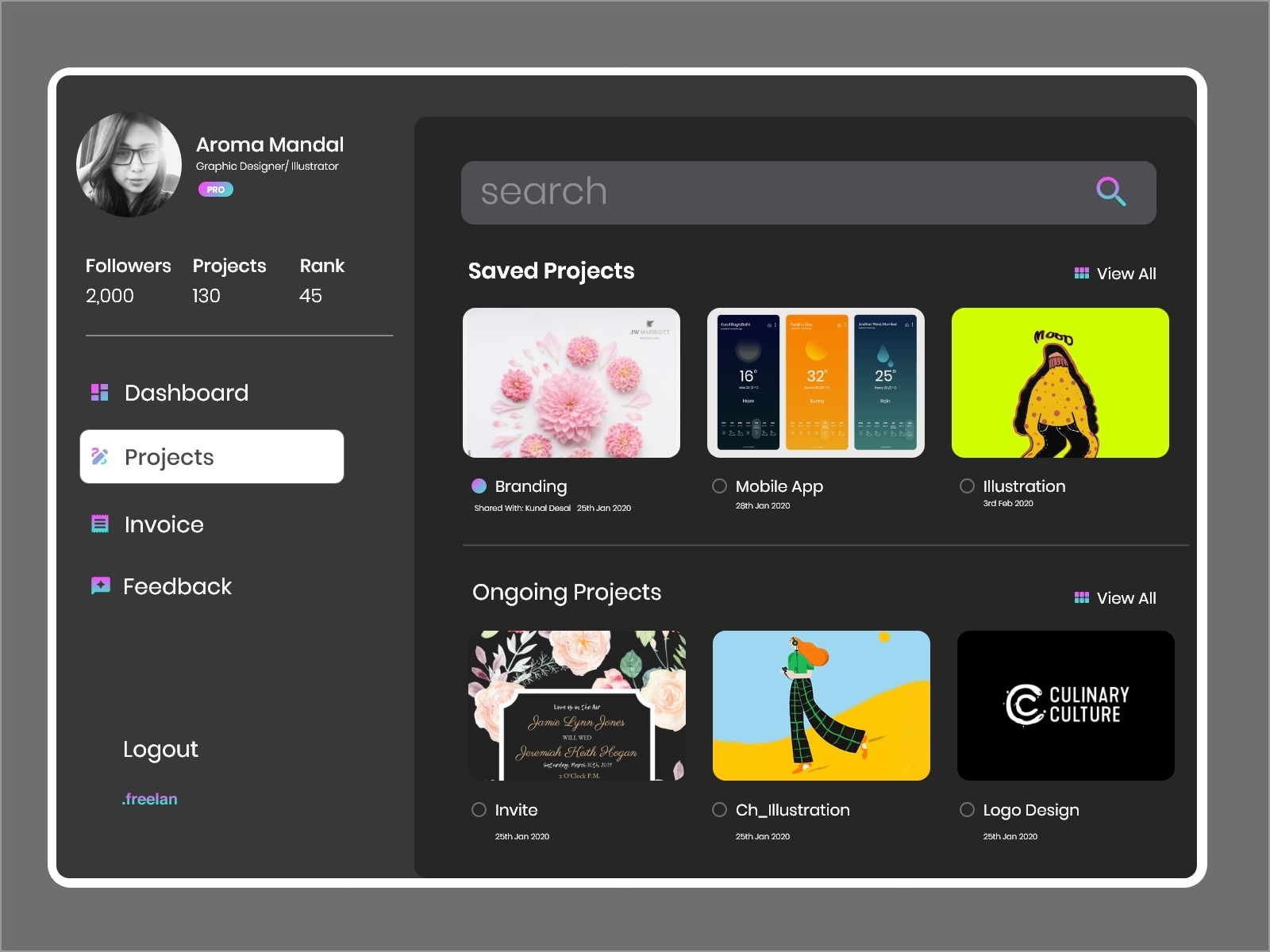A screenshot set against a gray background displays the user interface of a design dashboard for Aroma Mandel, a graphic designer and illustrator. Aroma, a young female with dark brown hair and black glasses, is identified in the upper left corner. Her profile details indicate she has 2,000 followers, has completed 130 projects, and ranks 45th. Below her profile, menu options are listed: Dashboard with a colorful icon, Projects highlighted in white, followed by Invoice, Feedback, and Logout options. The screen’s upper right corner features a search bar with the text “Search” in gray. The main section is divided into two parts: three saved projects and three ongoing projects, each displayed within individual boxes.